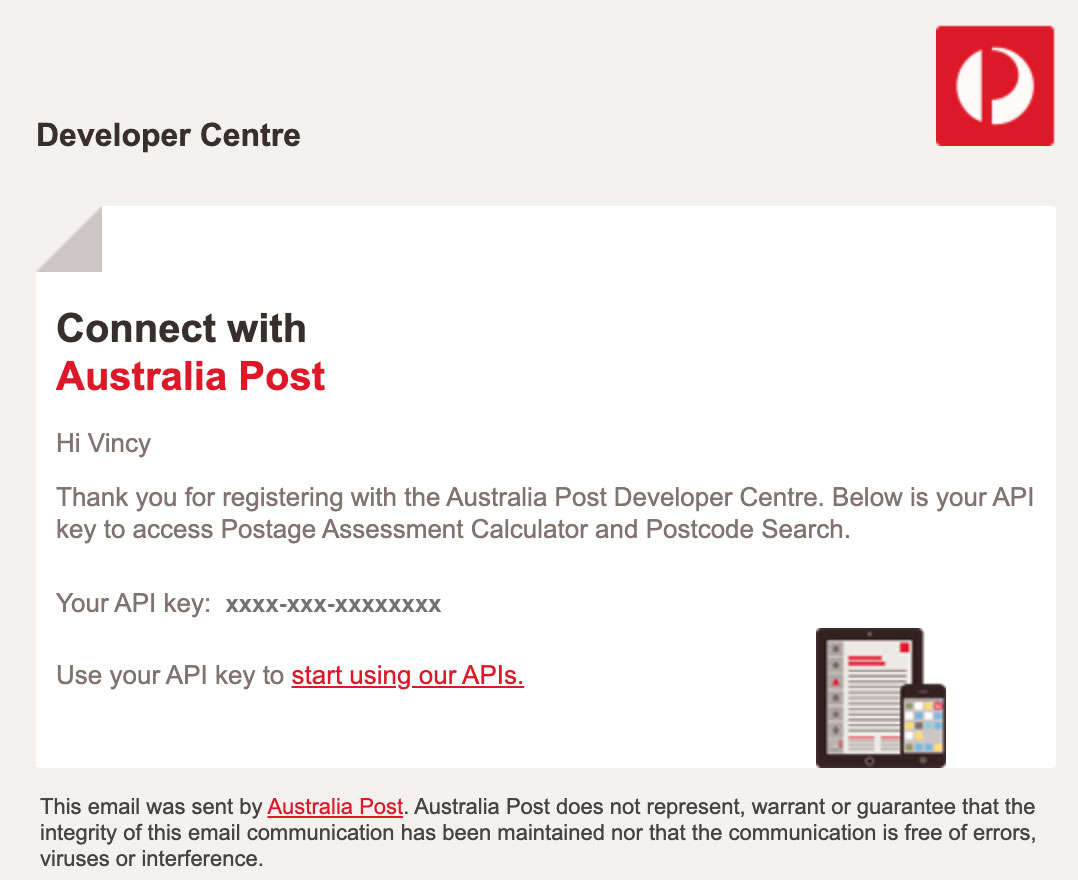The image is a detailed section of an email with a pale gray background and a landscape (sideways rectangle) orientation. 

In the top right corner, there is a red square featuring a distinctive white logo composed of a semicircle on the left and a swoosh on the right, forming a red "P" in the middle—this is the logo of Australia Post. 

In the top left, bold black letters spell out "Developer Centre," using the British spelling with “C-E-N-T-R-E.” 

Below this, a white rectangle spans the entire width of the screen. The top left corner of this rectangle appears folded over, showcasing a gray triangle. The text within the white rectangle reads:
- "Connect with Australia Post," where "Connect with" is in black and "Australia Post" is in bold red.

Beneath that, in a smaller non-bold font, it states:
- "Hi Vincy." (Spelled "V-I-N-C-Y")
- "Thank you for registering with the Australia Post Developer Centre."
- "Below is your API key to access Postage Assessment Calculator and Postcode Search."

Following this, the text reads:
- "Your API key:" followed by a string of characters represented as "X-X-X-X-X-X-X-X-X-X-X-X-X-X-X-X."

Another line instructs:
- "Use your API key to start using our APIs," where "Start using our APIs" is in bold red and underlined, indicating a clickable hyperlink.

In the bottom right corner, there is a simple cartoon-style illustration of a smartphone and tablet screen.

At the very bottom on the pale gray background, beneath the white text box in the center, a line of text reads:
- "This email was sent by Australia Post," with "Australia Post" in red and underlined, making it a clickable link.
- Adjacent to this, there is a disclaimer stating: "Australia Post does not represent, warrant, or guarantee that the integrity of this email communication has been maintained, nor that the communication is free of errors, viruses, or interference."